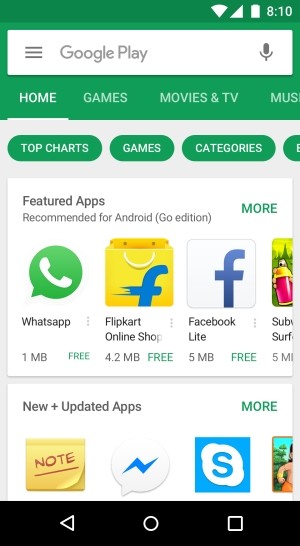The image features a screenshot of a Google Play Store page on an Android device. The top of the screen displays a dark emerald green status bar showing the Wi-Fi signal, cell signal, battery level, and the time, which reads 8:10. Below this, the header transitions to a lighter kelly green and includes a search bar with the text "Google Play," a microphone icon, and a menu icon represented by three horizontal lines.

Immediately under the header, in white text, are navigation options labeled "Home," "Games," "Movies & TV," and "Music." The main content area of the page features a gray background with green and white tabs labeled "Top Charts," "Games," "Categories," and a partially visible fourth tab.

A prominent white square section is dedicated to featured apps recommended for Android Go Edition. To the right of this section, the word "MORE" is written in green, capitalized text. Below this section, the graphics of the featured apps are displayed. The first graphic has a green background with a white telephone icon and the word "WhatsApp." The second graphic features a green and yellow shopping cart with a blue "F" and the text "Flipkart Online Shop." The third graphic shows a blue "F" representing Facebook, and a fourth partially visible app icon.

Further down, a section labeled "New and updated apps" shows another "MORE" option in green text. Highlighted apps in this section include the Skype logo and a white circle with a blue lightning bolt, though the latter's details are partially cut off.